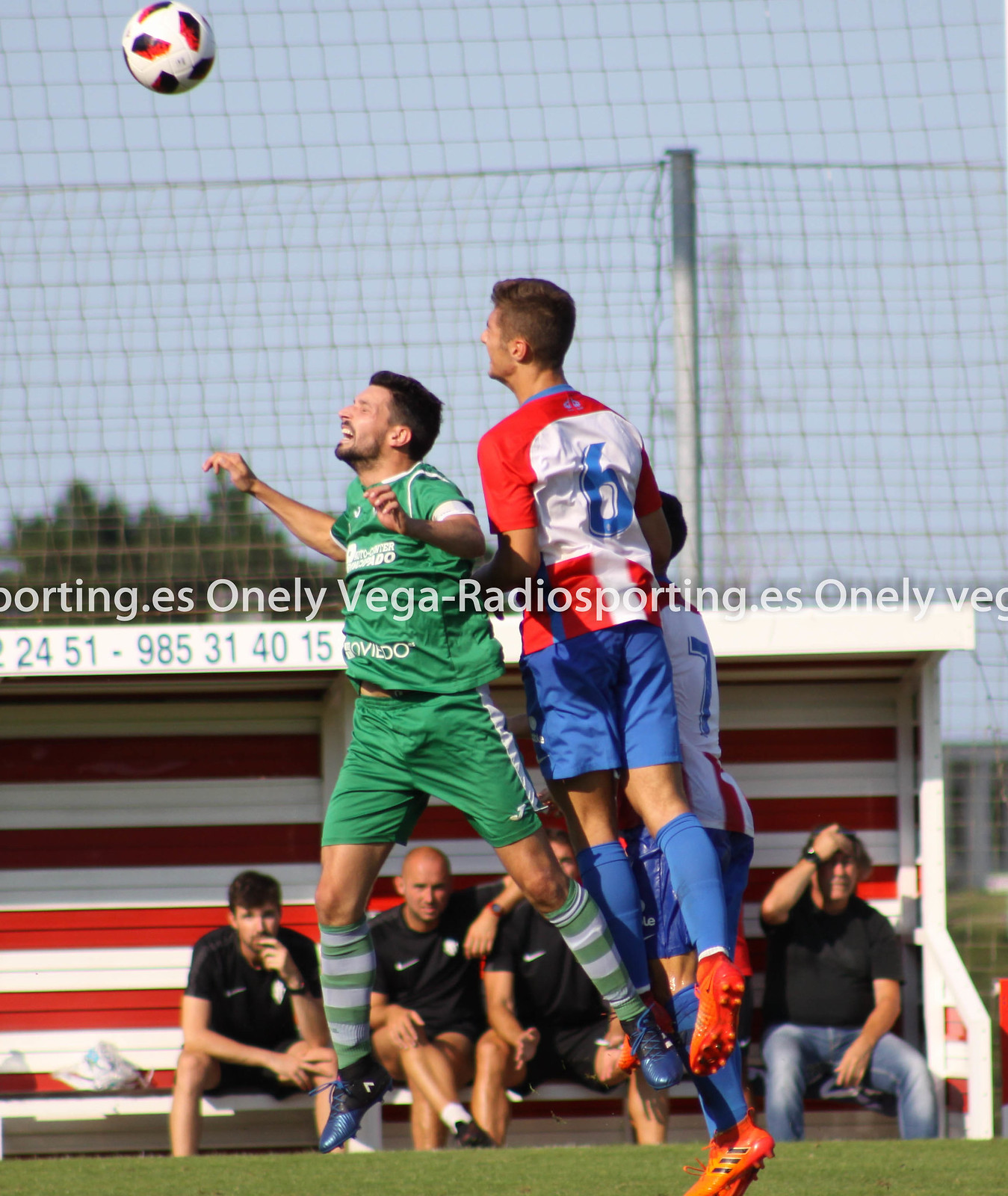In the photograph of a soccer match, three men are seen leaping into the air attempting to intercept a white soccer ball with red and black markings that is positioned in the upper left corner of the image. The man on the left is distinguishable by his green uniform, which includes a t-shirt and shorts with white trim, green and gray striped socks, and blue boots. His two opponents are clad in white shirts, red detailing, and blue shorts, sporting orange boots. In the background, a group of spectators in black shirts can be observed sitting on a bench within a white and red dugout. The setting is enclosed by a large net that stretches across a blue sky. Prominent text overlays the middle of the picture, likely reading "OneLeagueVegaRadioSporting.es," and repeats horizontally across the image.